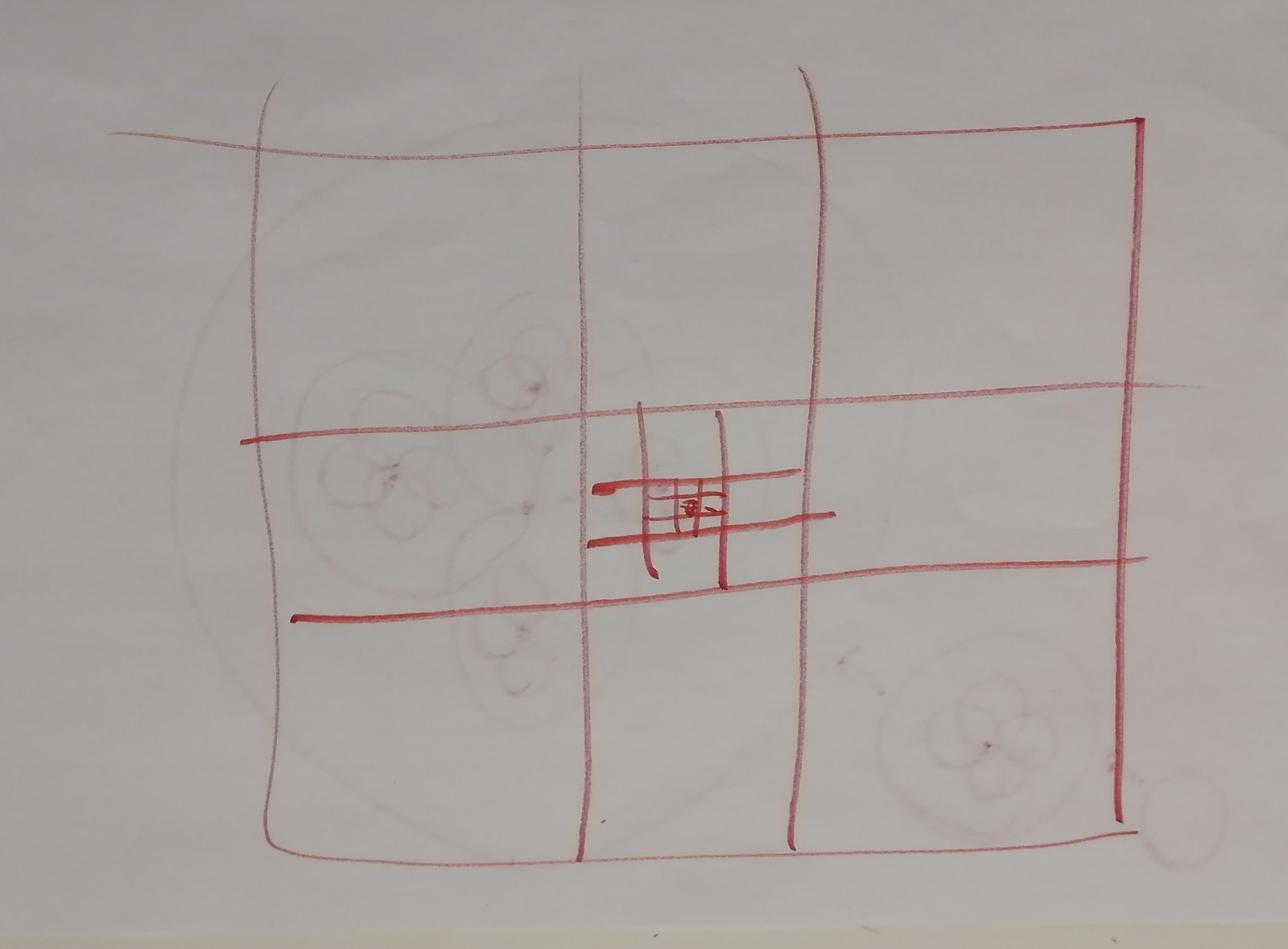This image appears to be a child's drawing on a large sheet of light-orchid colored paper. The drawing features twelve large red squares, which have been drawn somewhat carelessly, with lines that are uneven and sometimes extending beyond their intended boundaries. In the very center of these twelve large squares, there's a smaller grid of nine squares, reminiscent of a tic-tac-toe board. Inside the central square of this tic-tac-toe grid, another nine-square grid has been drawn, and in the middle square of this smallest grid, there is a red circle. The lines vary in intensity, with some being heavily marked in dark red and others appearing lighter and more delicate. The overall impression is one of a free-form, imaginative drawing, indicative of a young artist still mastering control over their materials and technique.